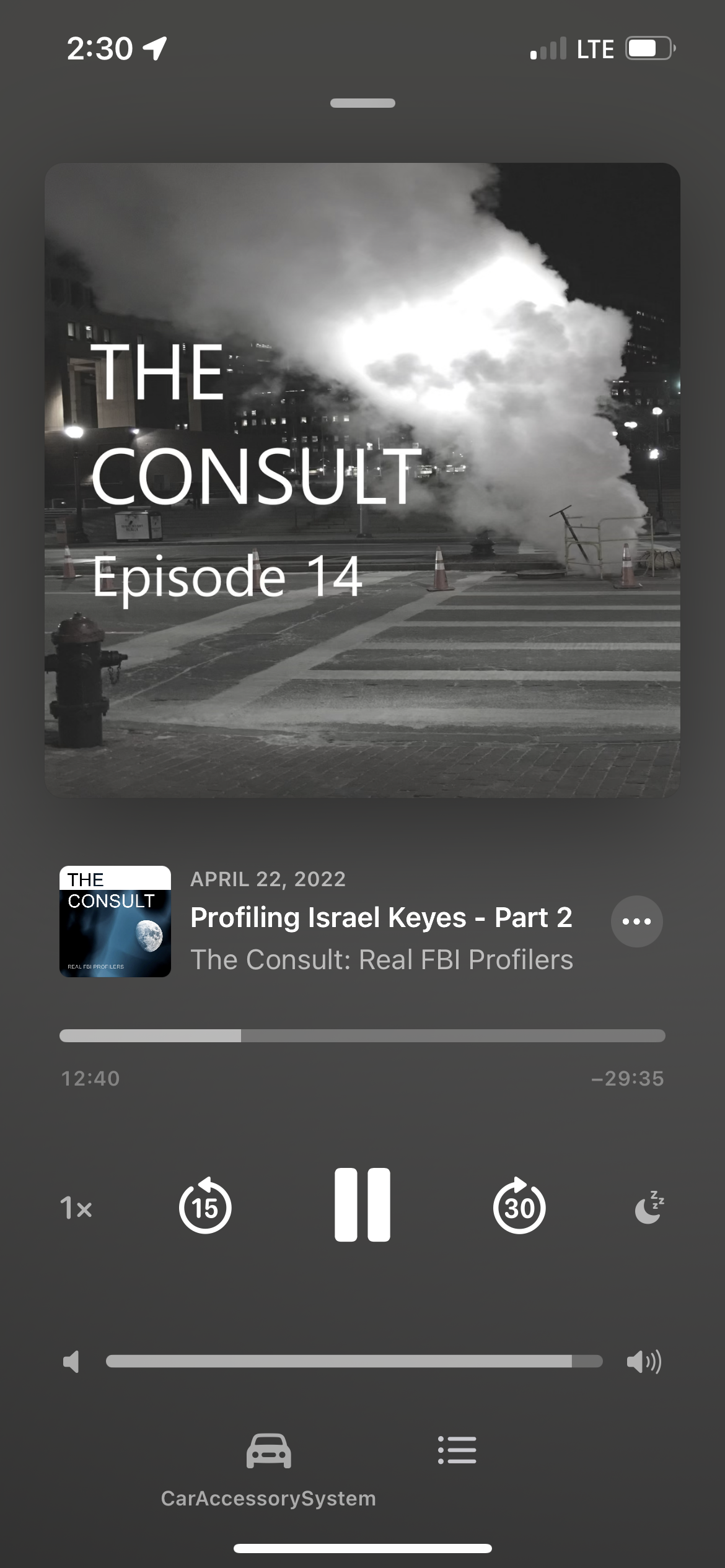This is a detailed description of a smartphone screenshot displaying a paused video titled "The Consult Episode 14." 

In the top left corner, the time reads 2:30, and the top right corner shows a battery level at approximately 75% with a single bar of cell service. The main focus is a black and white video still showing a street with a crosswalk, a fire hydrant, and rising white smoke in the background with a cityscape behind it. The video content is about "The Consult," specifically "Episode 14," profiling Israel Keyes, part 2, with a release date of April 22, 2022, hosted by real FBI profilers.

The video is paused at 12 minutes and 40 seconds, with 29 minutes and 35 seconds remaining. There are playback controls visible: options to speed up the playback, rewind 15 seconds, pause, and fast-forward 30 seconds. The volume is nearly at maximum. Additionally, a notification bar at the bottom indicates the phone is connected to a car accessory system.